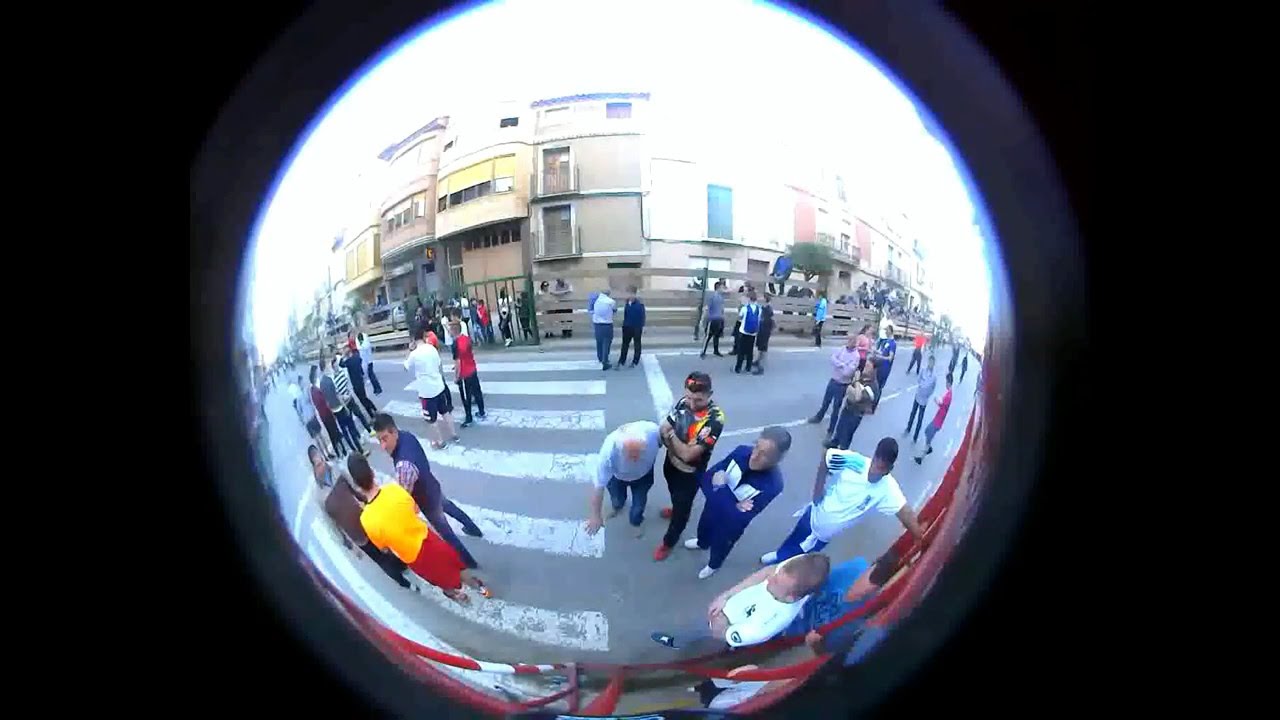Peering through a keyhole, the image captures a bustling urban street scene slightly distorted by a fisheye lens. The view, encircled by the keyhole's frame, centers on a black asphalt road segmented by a white crosswalk. Around 75 to 80 people populate the street, their varied poses suggesting animated conversations and interactions. Some are leaning against a red rail at the base of the keyhole, while others stand in groups or alone. No cars are in sight, amplifying the festive, pedestrian-dominated ambiance. Flanking the street are three- to four-story buildings, with onlookers peering from the sidewalks. The scene is brightly lit, indicating a daytime setting.